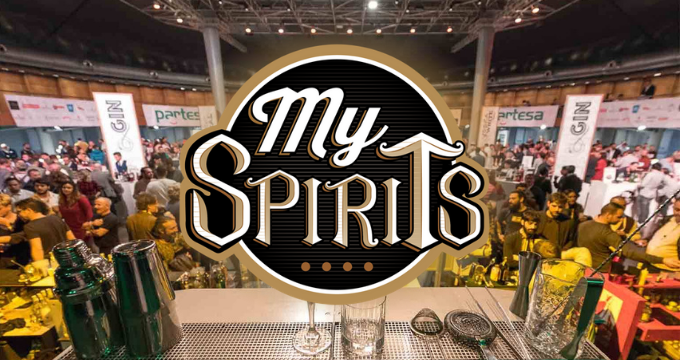The image depicts the interior of a large establishment, possibly a convention center or a grand bar area, bustling with activity. The setting reveals numerous people scattered throughout, clad in varied attire, with a notable woman in a red top on the left side. Central to the image, dominating the view, is a prominent, round logo labeled "My Spirits." This logo has a gold-tan outer ring, a white inner circle, and a black interior where the white, gold-outlined text "My Spirits" is prominently displayed, along with four reddish-tan dots beneath "spirits." Overhead, the ceiling features a complex metal rafter system housing extensive lighting apparatuses. On either side of the spacious interior, white banners with the word "Gin" in black text hang. Below the logo, a light gray table with silver barware hints at a drink-serving setting, suggesting perhaps a drink-tasting event or a themed bar area within this expansive venue. The area teems with vibrant colors including black, white, red, blue, yellow, gold, brown, and green, enhancing the lively atmosphere.